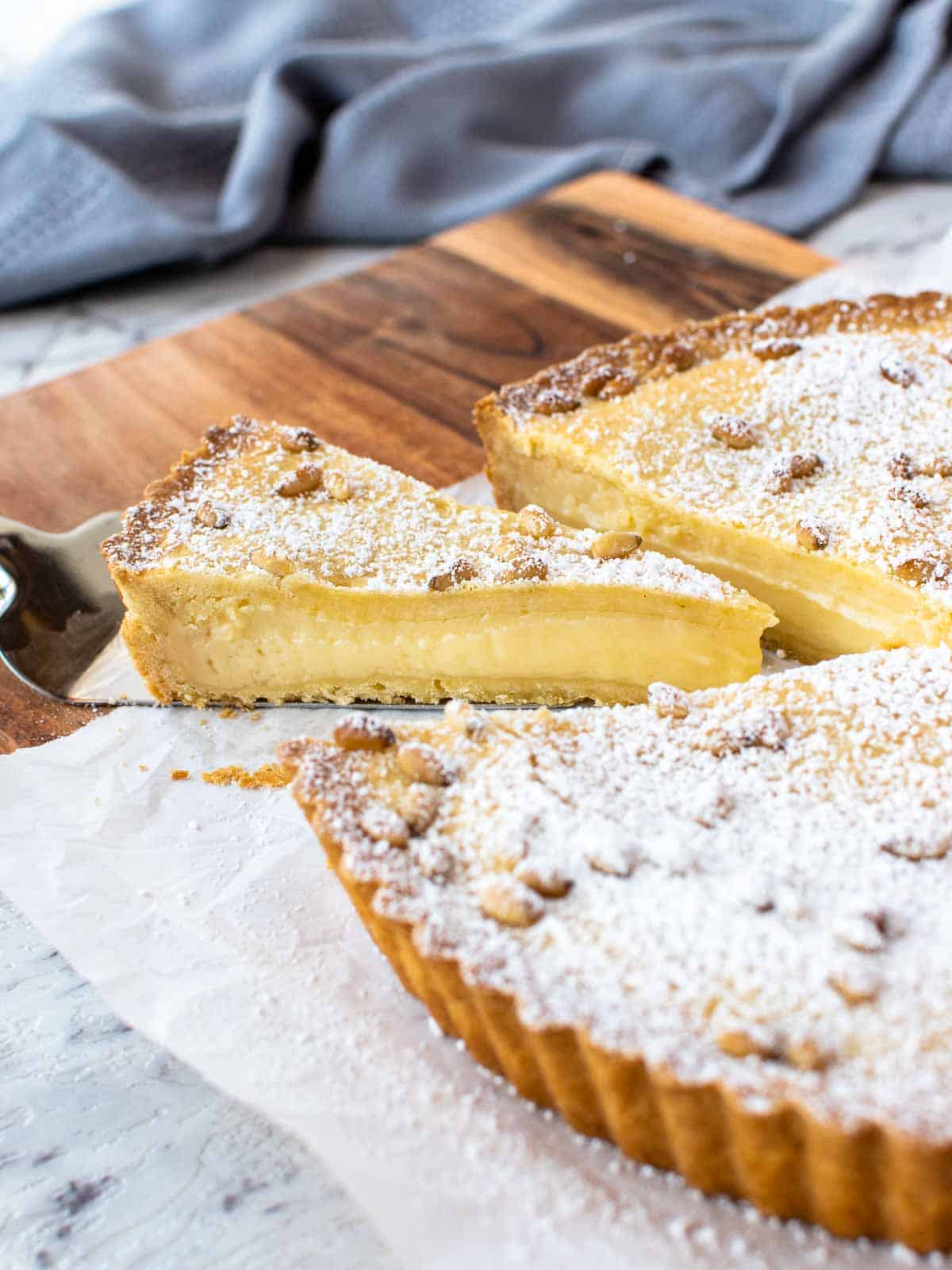This indoor photograph captures a meticulously presented pie, set on a large wooden cutting board layered with parchment paper. The pie, which has a golden-brown crust dusted with powdered sugar and garnished with chopped nuts, reveals a creamy yellow custard filling, possibly reminiscent of a custard pie or cream pie. One slice has been carefully removed and is balanced on a silver pie server, positioned to the left of the main dish. In the background, the kitchen scene includes a blue kitchen towel laid out on a countertop, adding a touch of color to the setup. Further back, a cabinet supports a wooden platter topped with a white cloth, enhancing the rustic ambiance of the setting.